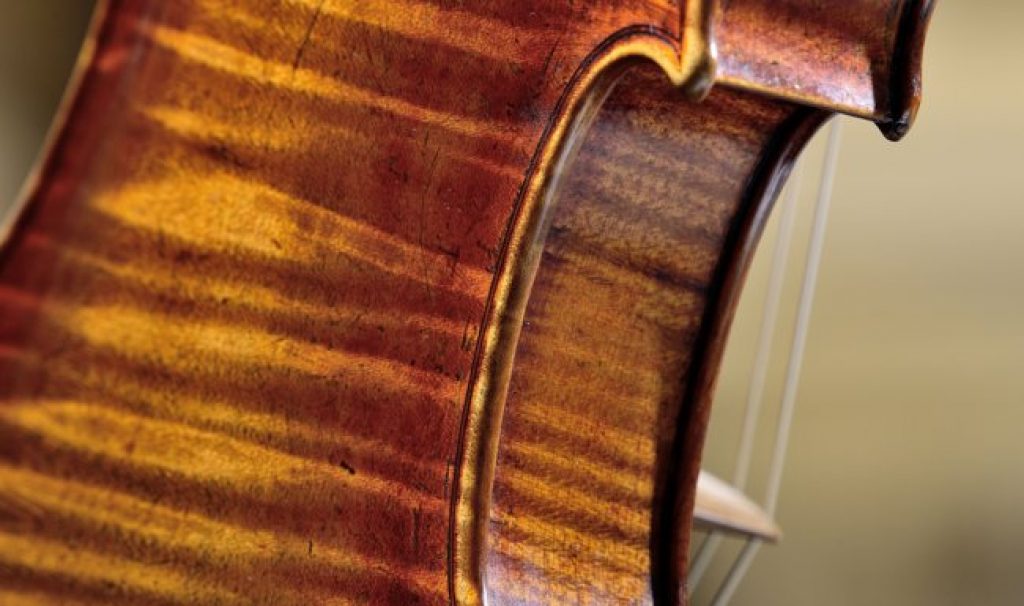A close-up photograph features the back of a well-used stringed instrument, likely a violin, fiddle, or viola, showcasing intricate woodwork. The wood appears medium to dark brown with distinctive, cigar-shaped bands in a yellowish-tan hue. Along the side, linear stripes varying from brown to golden brown highlight the craftsmanship. Small black scratches on the surface suggest it has been lovingly handled over time. The right side of the image includes the bridge and two white strings of the instrument, emphasizing its functional and aesthetic details. The blurred background, in shades of beige, gray, and white, ensures focus on the instrument's textured and colored wood, reinforcing the overall brown and earthy tones of the image.